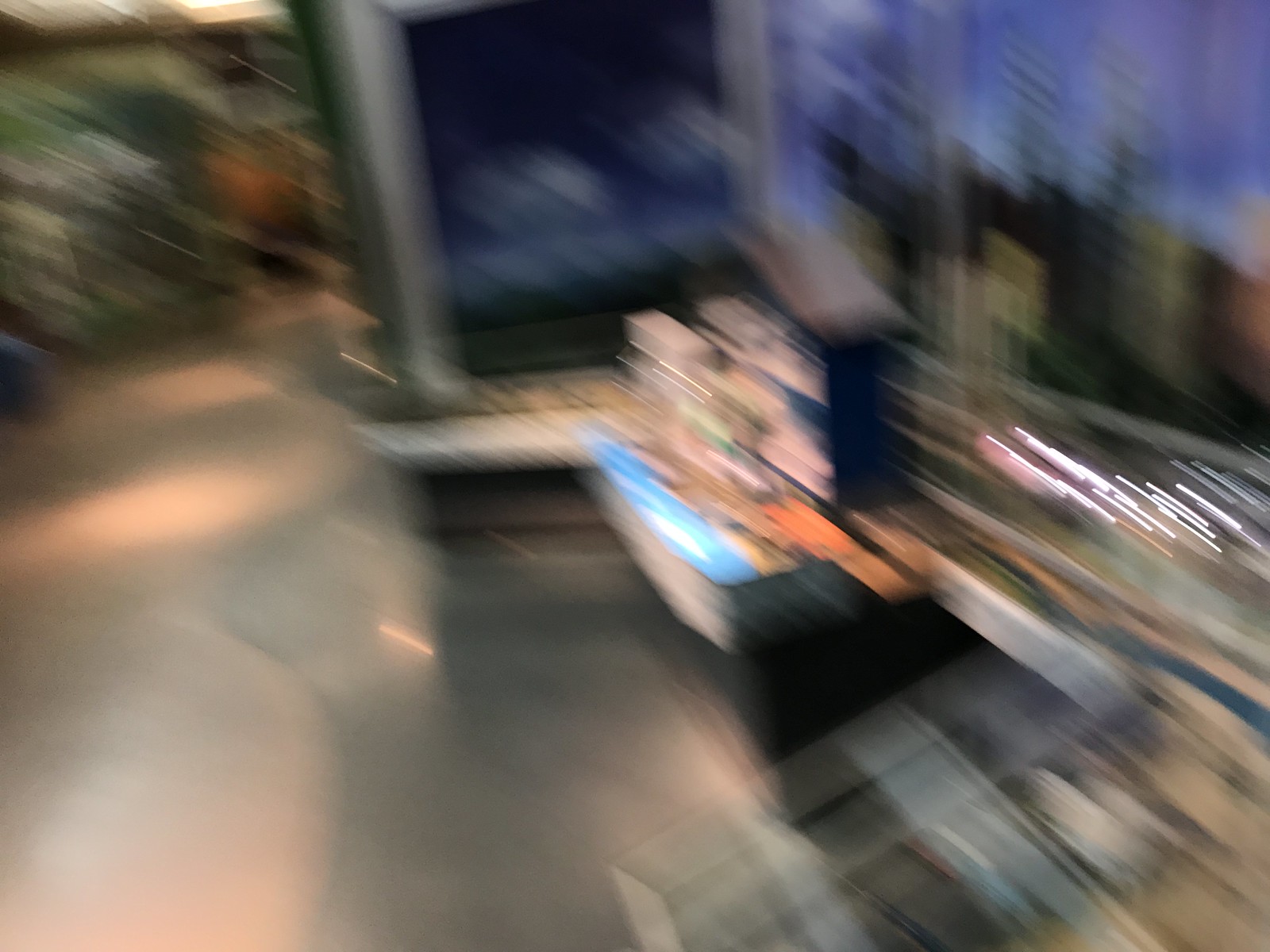A color photograph depicts a highly blurred scene, likely caused by camera movement or low light conditions. The image has streaks of light suggesting motion, creating a ghostly effect. At the center, there's a square or rectangular object that could be a sign or possibly a fireplace, resting on a pedestal. The floor, visible in the left portion of the image, is gray with reflective patches, implying it may be a polished surface. The rest of the scene remains indistinct due to heavy blurring.